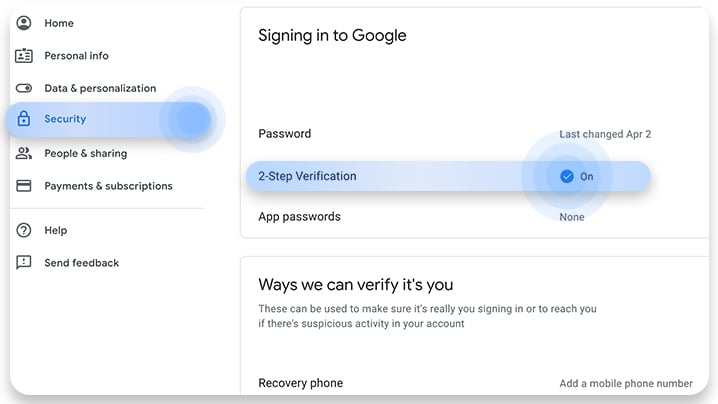This image depicts the "Security" section of a user's Google account settings. On the left-hand sidebar, starting from the top, there are several menu options including: Home (with an accompanying user icon), Personal Info, Data & Personalization, Security (the currently selected, highlighted in blue), People & Sharing, Payments & Subscriptions, Help, and Send Feedback.

On the right side of the image, there are two rectangular sections. The top section is titled "Signing in to Google." It displays the user's password status, indicating it was last changed on April 2nd, and shows that 2-Step Verification is enabled with no app passwords set. At the bottom of this section, it discusses "Ways we can verify it's you," emphasizing that these options are used for confirming the user's identity during sign-in or when suspicious activity is detected. The first option listed is "Recovery phone," with a prompt to add a mobile phone number to the right.